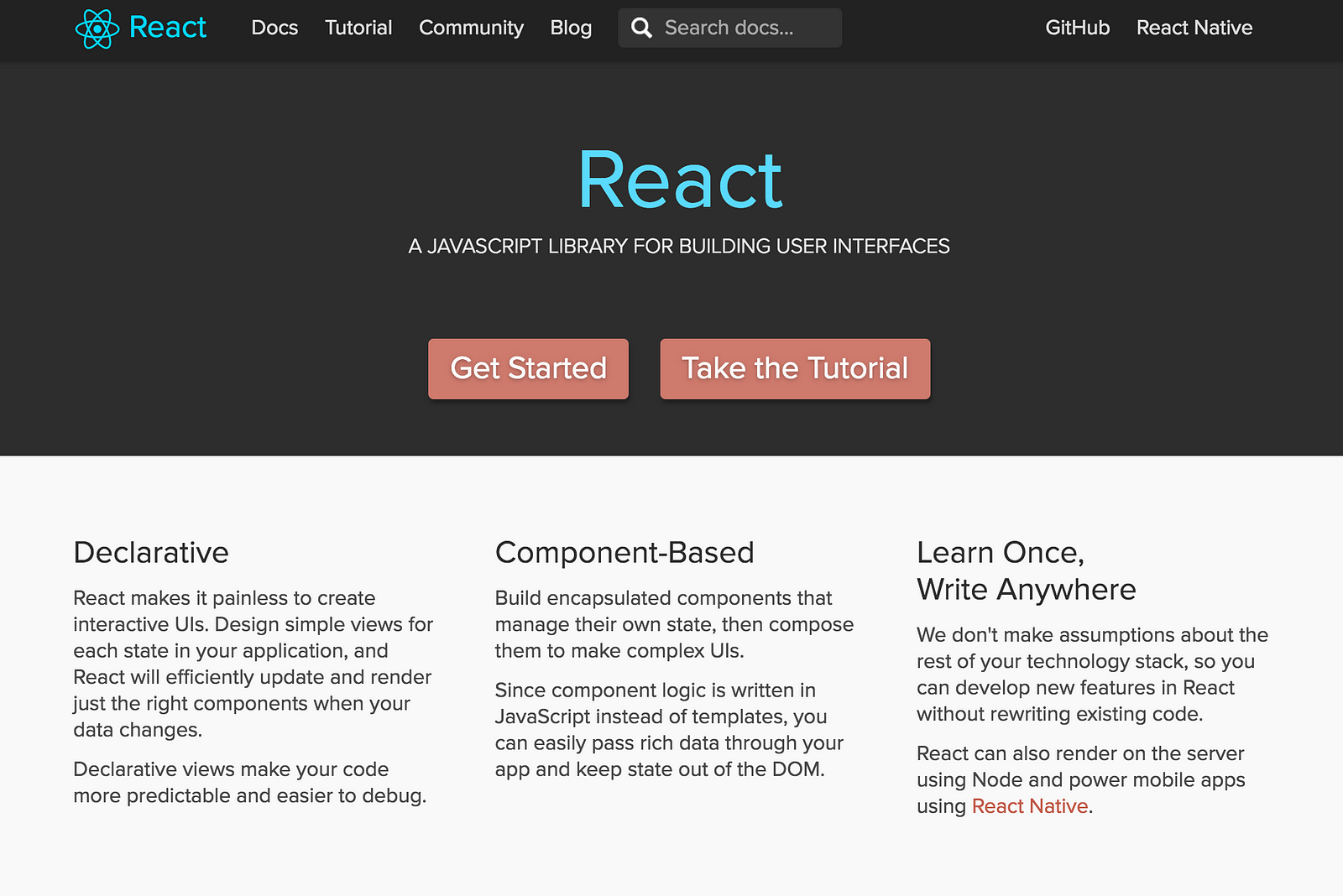The image displays the React web page. At the top left corner, the React logo prominently appears, indicating that this is an official page for React. The main navigation bar features categories such as "Docs," "Tutorial," "Community," and "Blog," providing easy access to various resources. To the right of the navigation bar, there is a search field labeled "Search Docs," enabling users to quickly find documentation.

In the top right corner, there are links to "GitHub," "React Native," and a tagline stating "React – A JavaScript library for building user interfaces." Below, large call-to-action buttons encourage users to "Get Started" with React or "Take the Tutorial."

The page highlights three core principles of React:
1. **Declarative:** The text explains that React simplifies the creation of interactive user interfaces by allowing developers to design simple views for each application state. React efficiently updates and renders the necessary components as data changes.
2. **Component-Based:** It promotes building encapsulated components that manage their own state, which can be composed to create complex user interfaces.
3. **Learn Once, Write Anywhere:** React avoids assuming specifics about the technology stack, enabling developers to add new features using React without needing to rewrite existing code.

Overall, the layout and content of the page are designed to introduce new users to React's features and guide them towards learning and adopting the library.